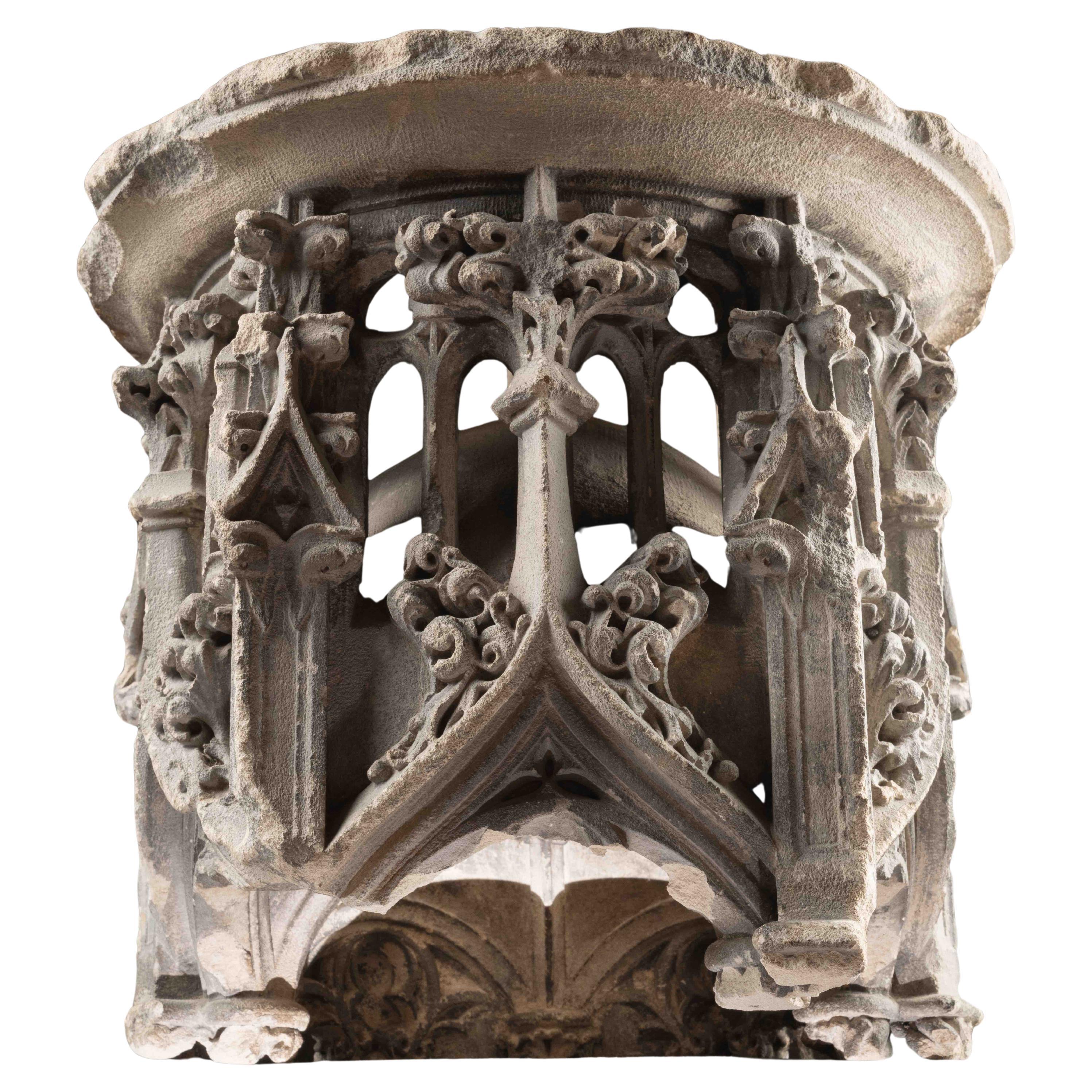The image depicts an ancient architectural structure, possibly a part of a column or tower, set against a white background. The cylindrical structure features a middle section adorned with intricate, abstract scrolled designs that are purely decorative, without representing any specific objects like animals or people. This ornate area is heavily weathered, with noticeable damages and large chunks missing, indicating its age and fragile state. The top of the structure is rugged and chipped, further accentuating its antique quality. The base has a more solid appearance with an open interior, revealing a bronze-colored creature’s head featuring eyes and a nose. The lighting appears to illuminate the structure from underneath, highlighting its Gothic design elements and giving it a slightly ethereal quality. The entire piece seems to evoke the grandeur of ancient Roman or Grecian architecture, with a possibility of it being a Doric temple fragment used in a Gothic church.